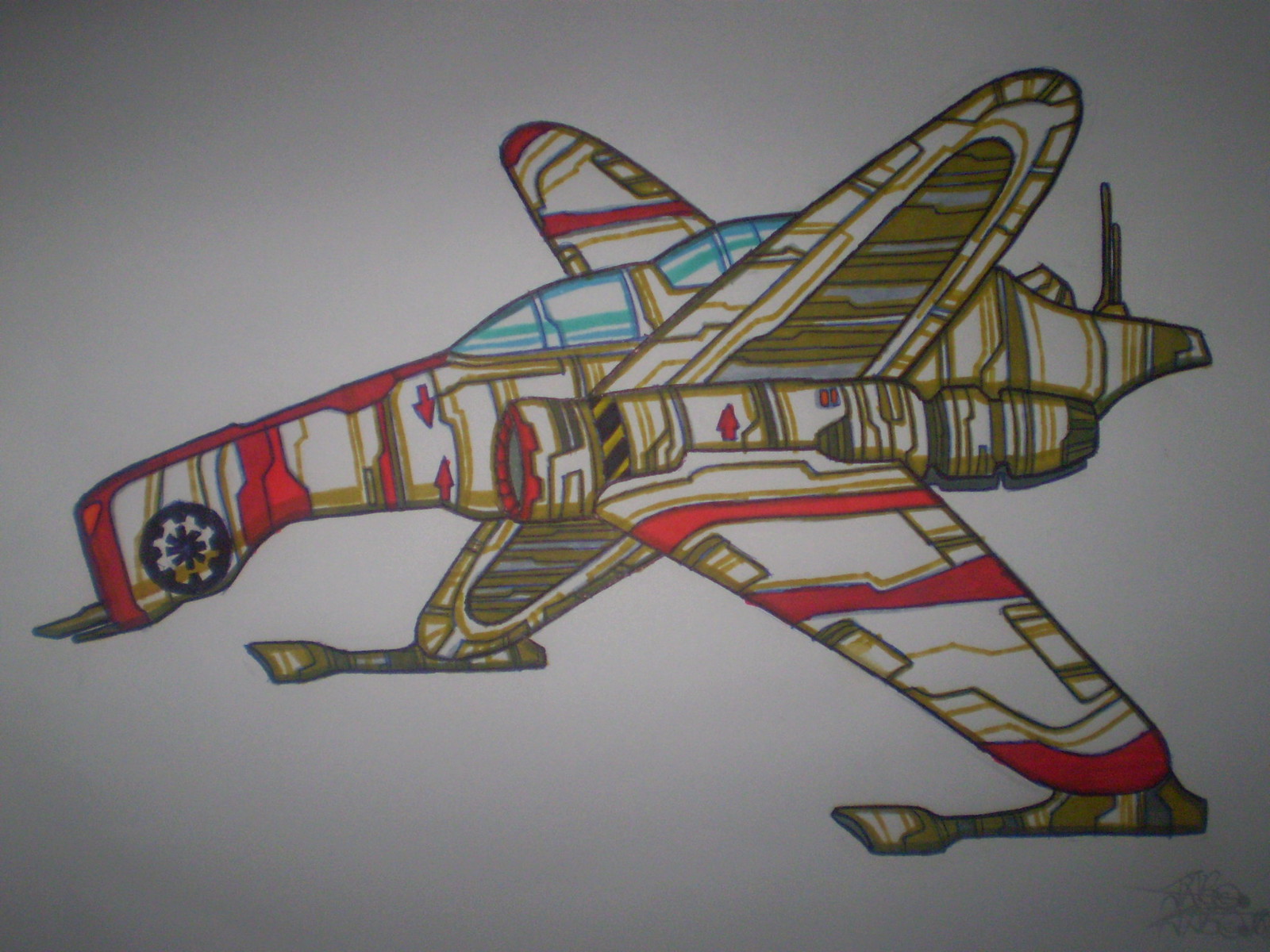The image depicts a colorful, intricately detailed decal, prominently featuring an X-Wing fighter from Star Wars, affixed to a wall, likely in a child's room. This X-Wing deviates from the classic color scheme, instead embracing a vibrant palette of yellows, browns, reds, and light blue. The underside of the wings are shaded with yellow and brown hues, while the upper sections and the area around the nose are highlighted in red, especially around the wing's curve. Notably, a black Rebellion symbol adorns the front nose. The drawing shows the X-Wing from an underside perspective, capturing details such as the dual light blue cockpit and droid seating areas and two antennae at the back. The artwork incorporates various line patterns, with sections of the plane left white, and includes distinctive elements like red-tipped wings and brown and green accents around the jet regions. The X-Wing's iconic guns and cannons are present, solidifying its identity despite the unconventional color choices.